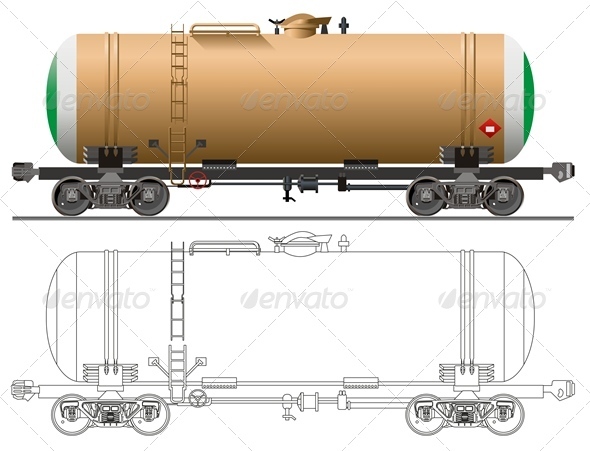The image features a detailed side view of a train tanker car, depicted in both color and architectural sketch formats. The top portion of the image presents a color rendition of the tanker's exterior, which predominantly features a gold body with green and white accents at both ends. The tanker, reminiscent of a large capsule, is mounted on a flatbed train car with visible gray wheels designed for railroad tracks. A ladder provides access to the top of the tanker, where a hatch and spout are visible, likely for inspection or access to its contents. Below the color image is a corresponding architectural sketch, which outlines the interior compartments of the tanker as well as the mechanical details of the train wheels. The entire image, set against a white backdrop, is faintly overlaid with a watermark that reads "Envato" in a pattern of diagonal lines forming a diamond-like design.